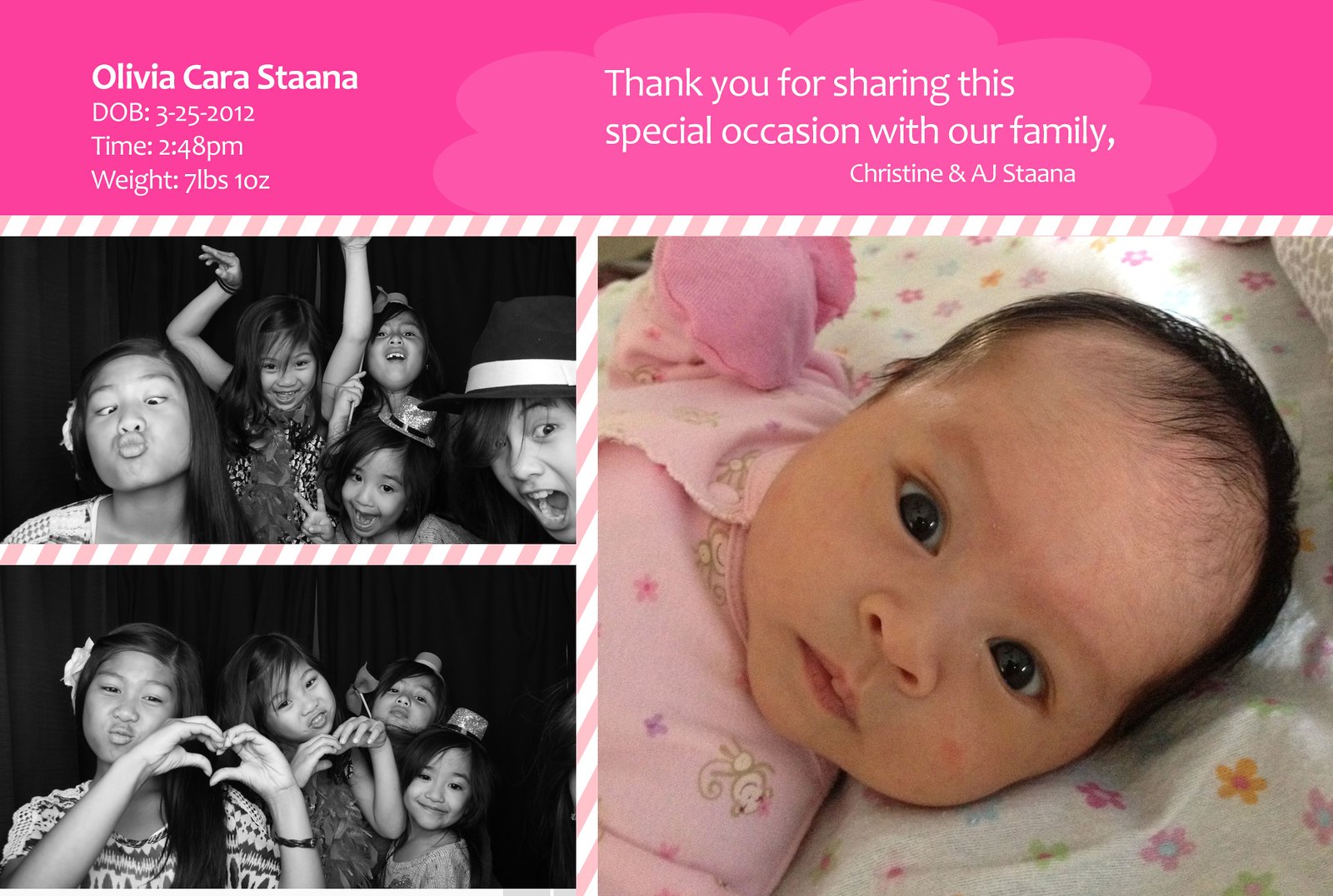The baby announcement for Olivia Cara Stana is a detailed and heartwarming graphic. At the top, a blue banner reads "Olivia Cara Stana" in white letters. Beneath it, pertinent birth details are listed: "Date of Birth: 3-25-2012," "Time: 2:48 PM," and "Weight: 7 pounds, 10 ounces." On the upper right, a touching message is displayed: "Thank you for sharing this special occasion with our family, Christine and AJ Stana."

The graphic is neatly divided by a pink and white striped border into two sections. The left side features two black and white photographs, one above the other. The top photo captures a group including four young girls and a boy popping his head in from the side, appearing to have fun. The bottom photo shows the same four girls making heart signs with their hands. On the right side, a larger color photo highlights the newborn baby girl, Olivia, wearing a pink onesie with designs. She has dark hair and dark eyes, further adding to the charm of the announcement.